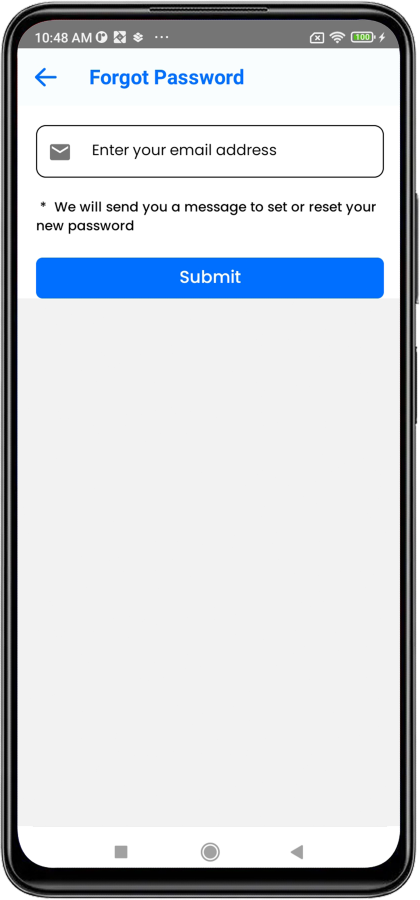The illustration depicts a smartphone with a dark gray frame displaying a webpage interface. The status bar at the top shows the time as 10:48 AM on the left, a fully charged battery icon at 100% on the right, and a WiFi icon. The screen itself has a very light gray background. Prominently in large blue bold font at the top center is the phrase "Forgot Password," accompanied by a left-pointing arrow to the left of the text.

Below this, a thin gray line outlines a rectangle containing a gray envelope icon on the left and the placeholder text "Enter your email address" in the same gray font. Underneath this rectangle, an instructional text reads, "We will send you a message to set or reset your new password" in gray font. Further down, a blue rectangular button labeled "Submit" in white font is prominently displayed.

At the bottom of the screen, the footer section stands out in white. In the center of this footer is a gray circle, flanked by a gray square on the left and a gray left-pointing triangle on the right.